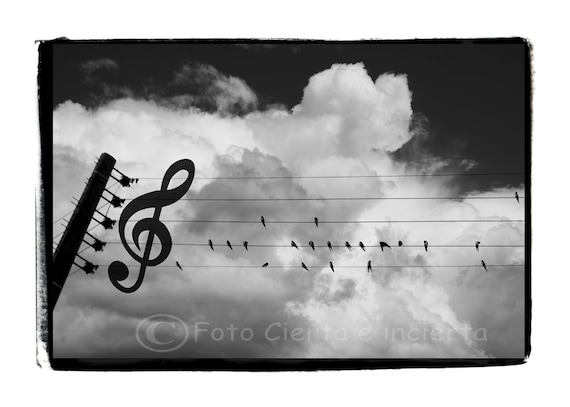This horizontally oriented image features a digitally edited, black and white photograph with artistic enhancements resembling a charcoal border. The central, realistic photograph depicts a dark sky with fluffy white clouds and a vertical telephone pole on the left, extending horizontally with five power lines. Perched along these wires are black silhouettes of birds, giving the impression of a musical staff. A large musical note, resembling a dollar sign, has been added to the left side of the image, transforming the scene into a visual representation where the birds appear as notes on a music scale. At the bottom of the image, a faint watermark in white lettering reads © F-O-T-O-C-I-E-R-T-A-E-I-N-C-I-E-R-T-A. The overall effect suggests that nature itself is composing a piece of music.